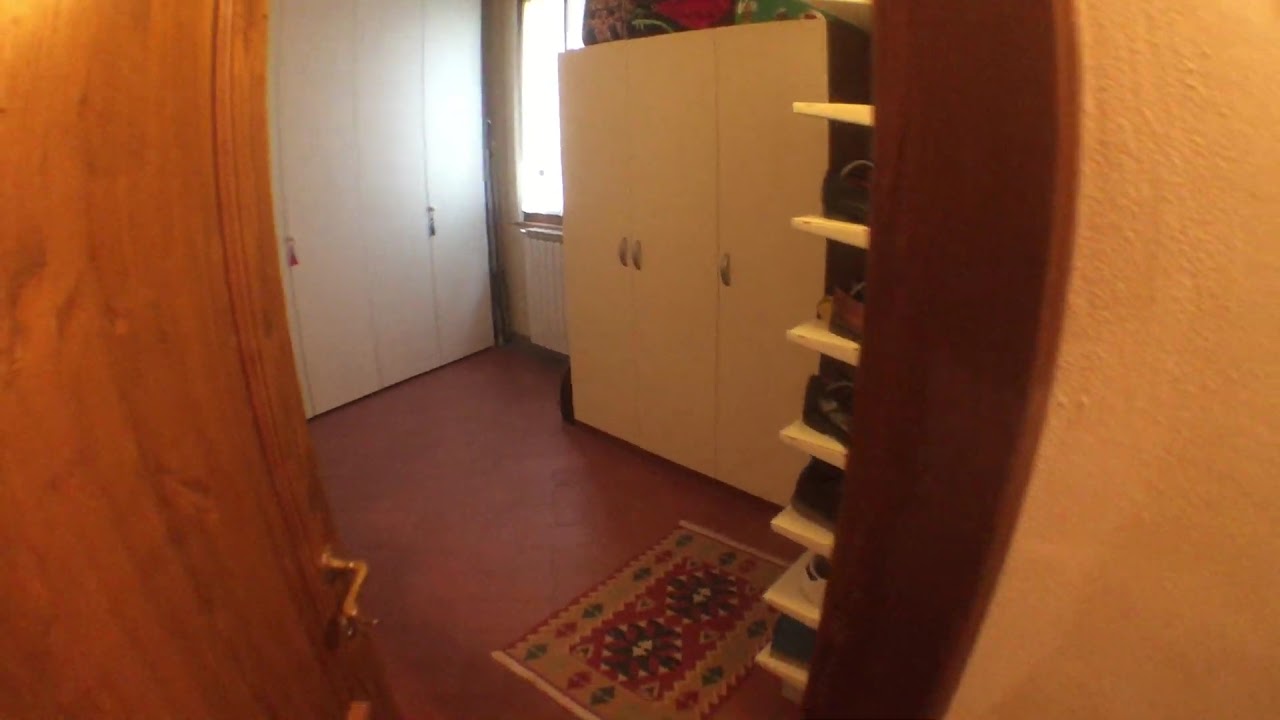This photograph, taken from a slightly unusual angle reminiscent of a fisheye lens effect, captures the interior of a neatly organized wardrobe room. The shot, taken from just outside the doorway, features a central brown door with a brass handle opening into the room. Inside, the focal points include two white closets on either side, both with silver pull handles. Positioned prominently against the left wall is a cabinet topped with various bags and suitcases. Off to the right, a series of seven shelves house an assortment of shoes, providing a glimpse into an organized collection. A window at the back allows sunlight to stream in, illuminating the woven rug on the floor which features rich tones of brown, red, green, and tan with triangular patterns. The room's walls and containers maintain a clean white color, contrasting with the reddish-brown floor. The photograph is devoid of any text or people, enabling full attention on the room's orderly setup captured in medium quality.